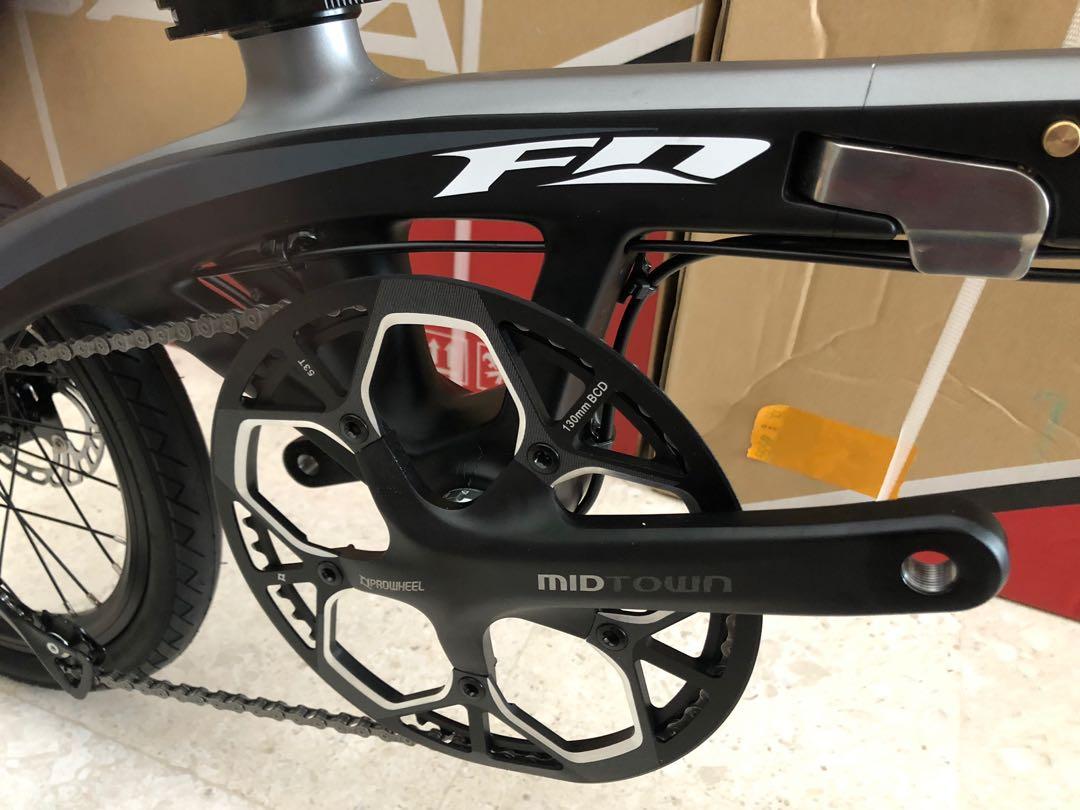The photograph captures a close-up view of the drivetrain mechanism of a brand new bicycle, freshly assembled. The image focuses on the crankset, the circular component around which the bike chain turns, but notably, the pedals have yet to be attached. The metal parts gleam with pristine, unblemished surfaces, showcasing the bike's newness. 

In the background, a cardboard box is partially visible, indicative of the bike's recent unpacking and assembly. On the right side of the crankset, the branding "Something Wheel Midtown" is clearly legible, suggesting a specific model or series. Additionally, the initials "FD" are marked in a stylish white font on another part of the bike. 

The bicycle sports a matte black finish, exuding a modern and sleek aesthetic. The rear tire is just barely visible, hinting at the overall structure of the bike. The crankset is marked with "130 millimeter BCD," a technical specification for the bolt circle diameter. The background box features some branding in white, black, and red against the standard brown cardboard, but its details are not entirely distinguishable. The scene suggests an ongoing assembly process of a high-quality bicycle, spotlighting its detailed craftsmanship and design elements.